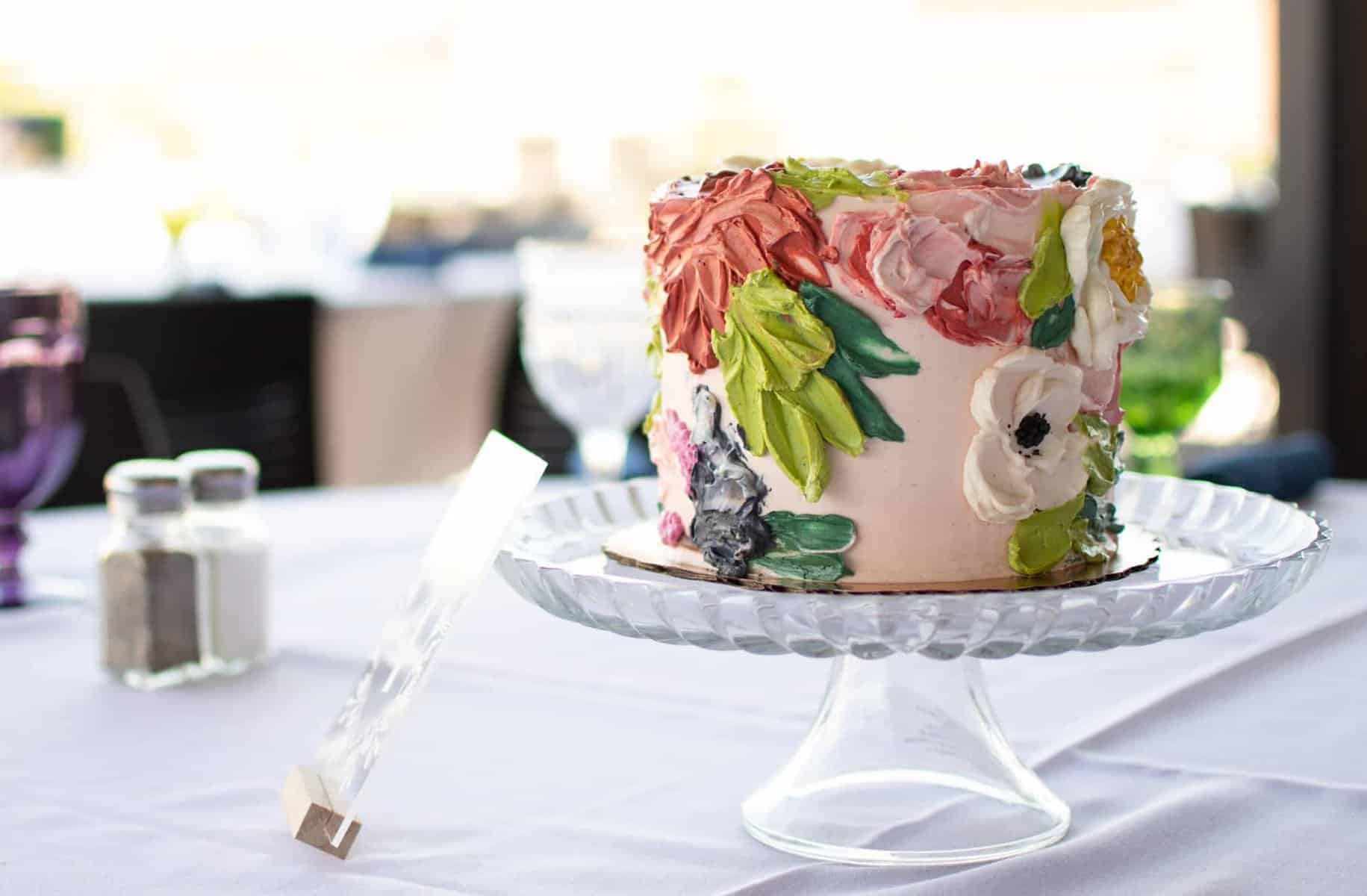This color photograph, captured in landscape orientation, showcases an elegantly decorated multi-layered cake. Positioned gracefully on a glass cake stand with a transparent foot, the cake stand rests atop a white tablecloth, which exhibits visible creases from prior folding. In the background to the left, a slightly out-of-focus pepper shaker and salt shaker add a subtle domestic touch to the scene. Additionally, a plexiglass holder leans against the cake plate, tilted away from the viewer.

The round cake itself is a masterpiece, adorned with smooth, pale pink frosting. The delicate yet vibrant decorations feature an array of flowers and leaves crafted with broad brush strokes. These floral embellishments display a rich palette of dark green, light olive green, pale pink, deeper pink, and purple hues. Notably, the cake remains uncut, preserving its pristine and artful appearance.